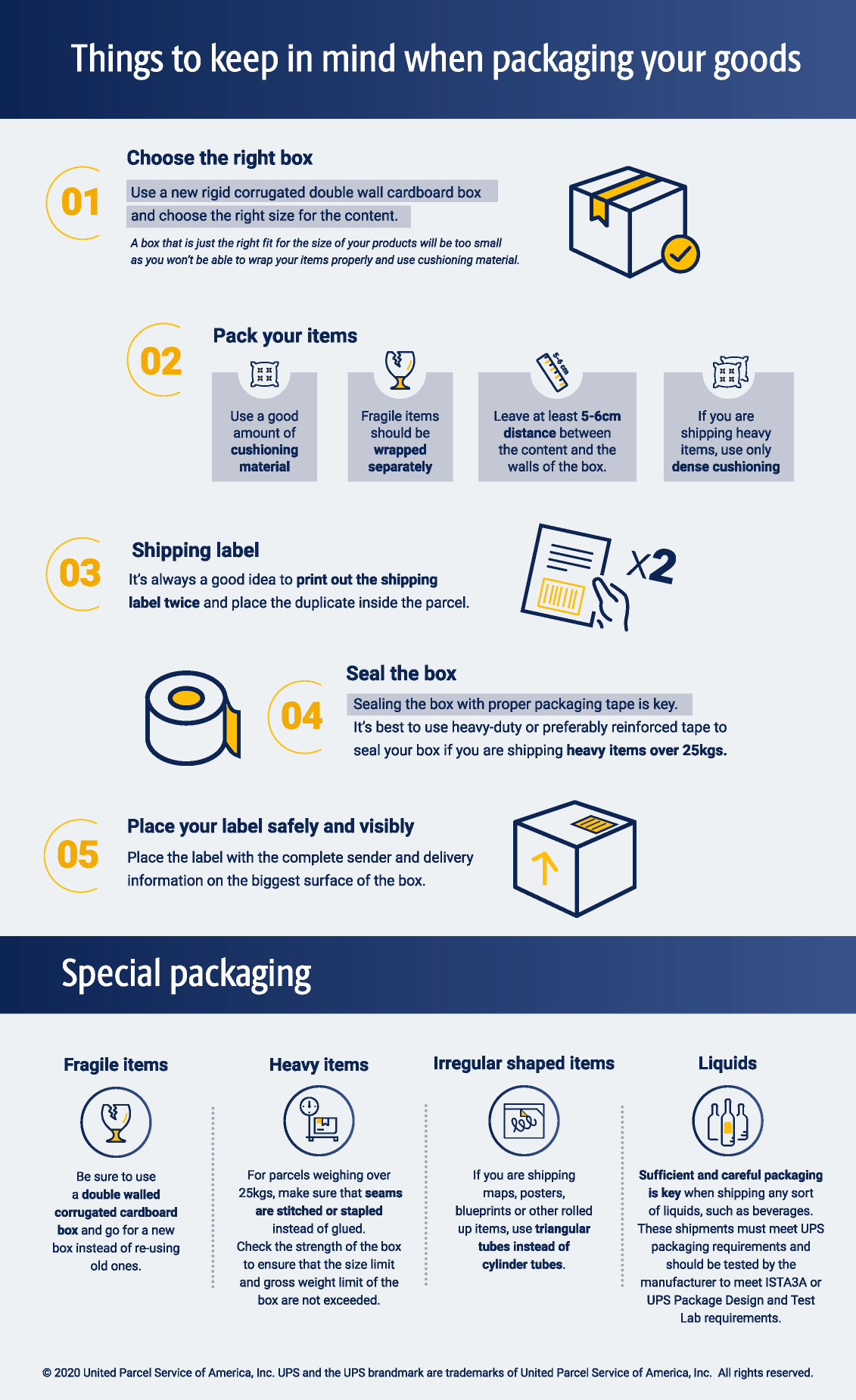This instructional poster, prominently featuring blue and gray tones with orange highlights, is aimed at guiding workplace staff on proper packaging techniques. Titled "Things to Keep in Mind When Packaging Your Goods," the poster outlines a five-step process:

1. **Choose the Right Box:** The poster underscores the importance of selecting an appropriate box, including a visual aid of a box.
2. **Pack Your Items:** Details and tips are provided, along with icons, advising on proper cushioning and ensuring a 5-6 cm space between contents and box walls. Fragile items should be wrapped separately.
3. **Create the Shipping Label:** The importance of printing the label twice is emphasized, with an illustration of someone holding a label marked "x2."
4. **Seal the Box:** Instructions include using proper packaging tape for secure sealing.
5. **Place Your Label Safely and Visibly:** An orange arrow points to the top of a box where a shipping label should be placed.

Below these steps, the poster elaborates on special packaging requirements for different types of items:
- **Fragile Items:** Use double-walled corrugated cardboard boxes.
- **Heavy Items:** For parcels over 25 kg, seams should be stitched or stapled.
- **Irregular Shaped Items:** Use triangular tubes for items like maps and blueprints.
- **Liquids:** Ensure sufficient and comprehensive packaging that meets UPS packaging requirements and has been tested to ISTA 3A standards.

The bottom of the poster contains the copyright information for UPS, reminding that the "UPS" and the "UPS trademark" are registered trademarks of United Parcel Service of America, Inc.